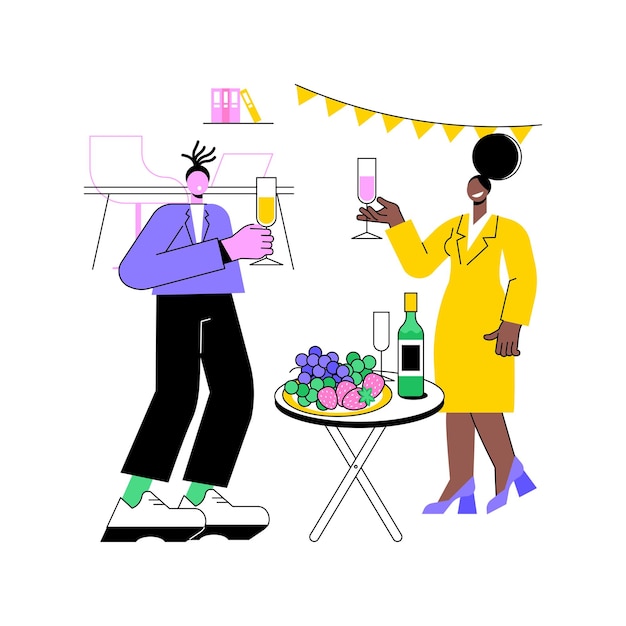This illustrated image, set against a white background, depicts a stylized, pop art-esque scene featuring a man and a woman with exaggerated proportions. Both individuals have disproportionately small heads compared to their bodies. 

On the left, the man has pinkish-purple skin and black dreadlocked hair tied up, complemented by a tiny beard. He dons a dark blue or purple jacket, black pants, green socks, and white shoes. In his hand, he holds a wine glass filled with yellow liquid.

To the right, the woman sports a prominent afro tied into a big bun atop her long, slender neck. She has brown skin and is dressed in a bright yellow, one-piece business dress that reaches her knees, paired with blue high heels and a tiny black choker. She holds a wine glass with purple liquid.

A small, round white table, supported by two crossed legs, sits between them. The table features a bottle of wine with a yellow cork, an empty glass, and a platter of grapes and strawberries. Above them, a banner made of little yellow triangles is strung up like festive decor. In the background, there is a chair and a small shelf with books, adding to the scene's ambience.